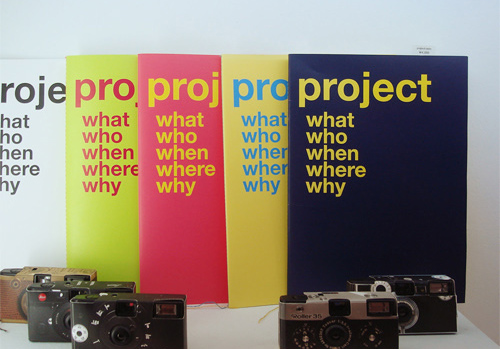The photograph features a white table with five disposable or instant cameras of various designs. From left to right, two cameras are black, while the remaining three are a mix of black and silver. Behind these cameras are five colorful booklets leaning against a white wall. The booklets are arranged in the following color order: white, lime green, pink, yellow, and dark blue. Each booklet has text in contrasting colors, with "project" written at the top and the words "what, who, when, where, why" listed below in lowercase letters.